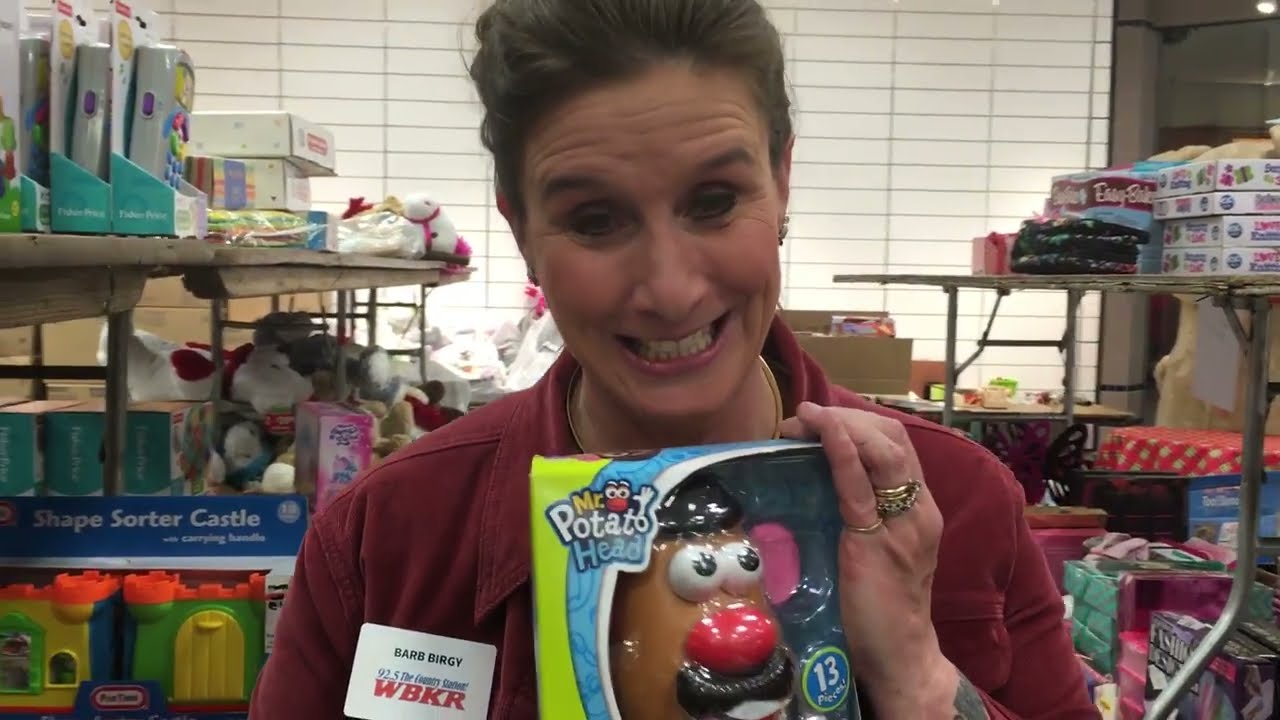The photograph captures an indoor scene, likely a toy store or warehouse, characterized by numerous shelves that are packed with disorganized toys, boxes, and stuffed animals. Situated centrally in the image is a Caucasian woman with tawny brown hair, which is brushed back and possibly tied into a ponytail or bun. She has a distinctive cheerful expression on her face as she looks at the camera, her head tilted to the side, eyebrows raised, and eyes outlined with eyeliner. She possesses dark blue eyes and is making a funny, closed-lip smile, indicative of her mid-speech.

She is attired in a red, button-down, collared shirt with a name tag that partially reads "B-A-R-B," suggesting her name is Barbara. She holds a boxed Mr. Potato Head toy from the Toy Story series, still in its official packaging. The background reveals a somewhat cluttered environment with shelves on either side and a large table strewn with various toys, emphasizing the setting's disorganized nature. Additional rooms can be glimpsed through a distant doorway on the right, and overhead lights illuminate the scene.